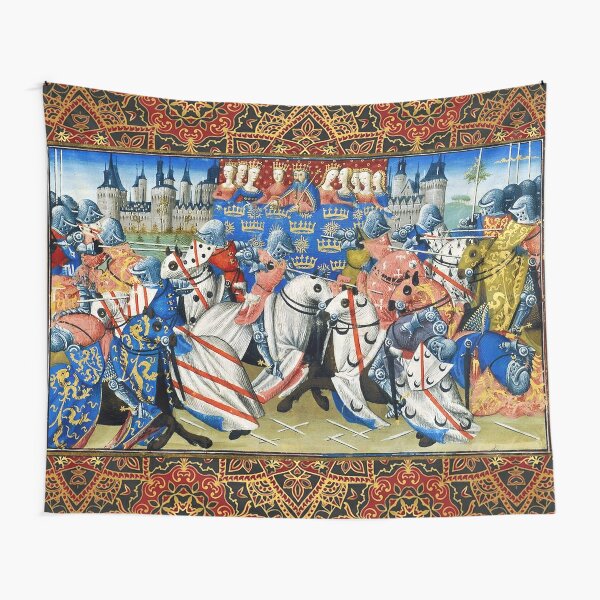The artwork is a nearly square tapestry pinned at each of the top corners onto a stark white wall. The scene depicted is a vibrant and detailed image from the Tournament of Camelot featuring a dynamic array of jousting knights on horseback. Each horse is adorned with distinctively colored and patterned blankets: one black horse wears a white sheet with black crescent moons, another dons a plain white sheet, while others feature patterns like black polka dots on white, red stripes on white, and blue with gold designs. There is also a horse with a yellow blanket and another with a gold one, alongside a striking pink-blanketed horse.

In the bustling foreground, knights clad in helmets and variously hued outfits brandish metal javelins, engaged in multiple jousts. The background showcases an opulent white castle with blue rooftops, framed by an intricate border adorned with gold, red, and black symbols. Above the tournament, the king sits prominently in a grandstand draped in blue fabric with gold crowns, flanked by nine women – four to his left and five to his right. These figures are partially blocking the view of the castle, adding layers of depth to the scene.

The tapestry's lower section displays the intricate details of the jousting grounds, which feature a light brown surface crisscrossed with white lines. Notable elements in the scene include the depiction of stylized bird heads and shields, adding to the rich and ornate quality of this historical tapestry.